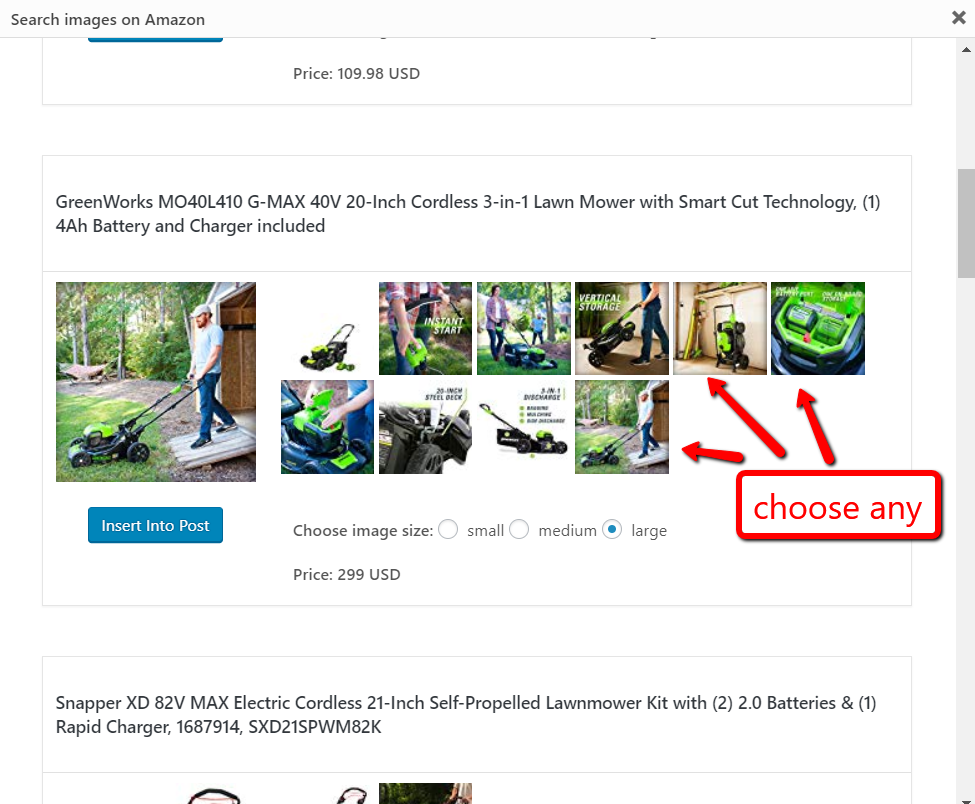This is a vibrant image of a webpage displaying lawnmowers available for purchase. The primary section focuses on a product titled "GreenWorks MO40L410G Max 40V 20-Inch Cordless 3-in-1 Lawn Mower with Smart Cut Technology." This product is priced at $109.98 USD, highlighted in blue with an 'X' button to remove it. Below the header, there's a small, Photoshopped image showing the lawnmower, and adjacent to it, a blue rectangle button with white text says "Insert into Post." 

Additionally, there's a red rectangle with three arrows labeled "Choose any," pointing to various product images. An option to select image size is also displayed, with "Large" selected and shaded in blue, indicated by a circle in front of each size option. 

Below the primary section, there's another product listing for the "Snapper XD 82V Max Electric Cordless 21-Inch Self-Propelled Lawn Mower Kit," priced at $299.99 USD. This listing includes details indicating the kit comes with two batteries and a rapid charger, noted in parentheses.